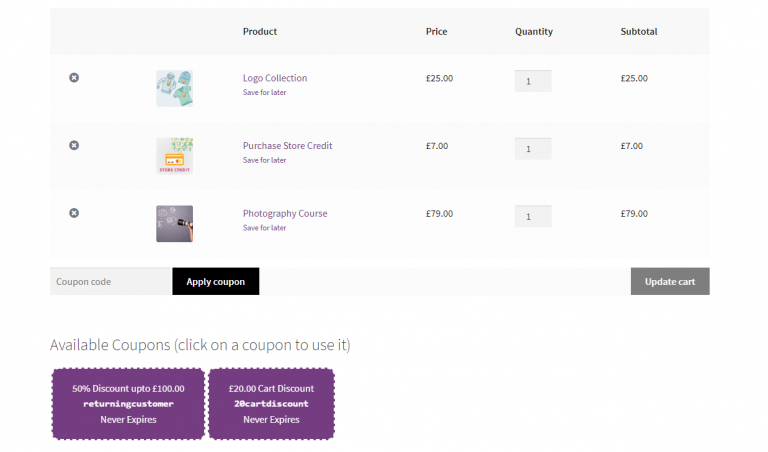The image displays a portion of a shopping cart interface, characterized by distinct sections and detailed information for each item. At the top, a gray bar separates the header from the main content. Below this header, the layout is divided into multiple columns.

The first segment under the header features an itemized list divided into three main rows, each representing a different product available for purchase, likely related to coursework. The leftmost section begins with a space that includes an 'X' button for removing items, followed by three entries: "Logo Collection," "Purchase Store Credit," and "Photography Course," each accompanied by a "Save for Later" option.

Moving to the right, the next column denotes the price of each listed item: $25 for the Logo Collection, $7 for the Purchase Store Credit, and $79 for the Photography Course.

The subsequent column specifies the quantity for each product, set at 1 by default, with editable boxes available for adjusting the quantity.

The rightmost column indicates the subtotal for each item, which are $25, $7, and $79 respectively. 

At the bottom of the interface, there is a button allowing users to apply a coupon or update their cart. The overall design is structured to facilitate easy management of selected products, including options for quantity adjustment and item removal.